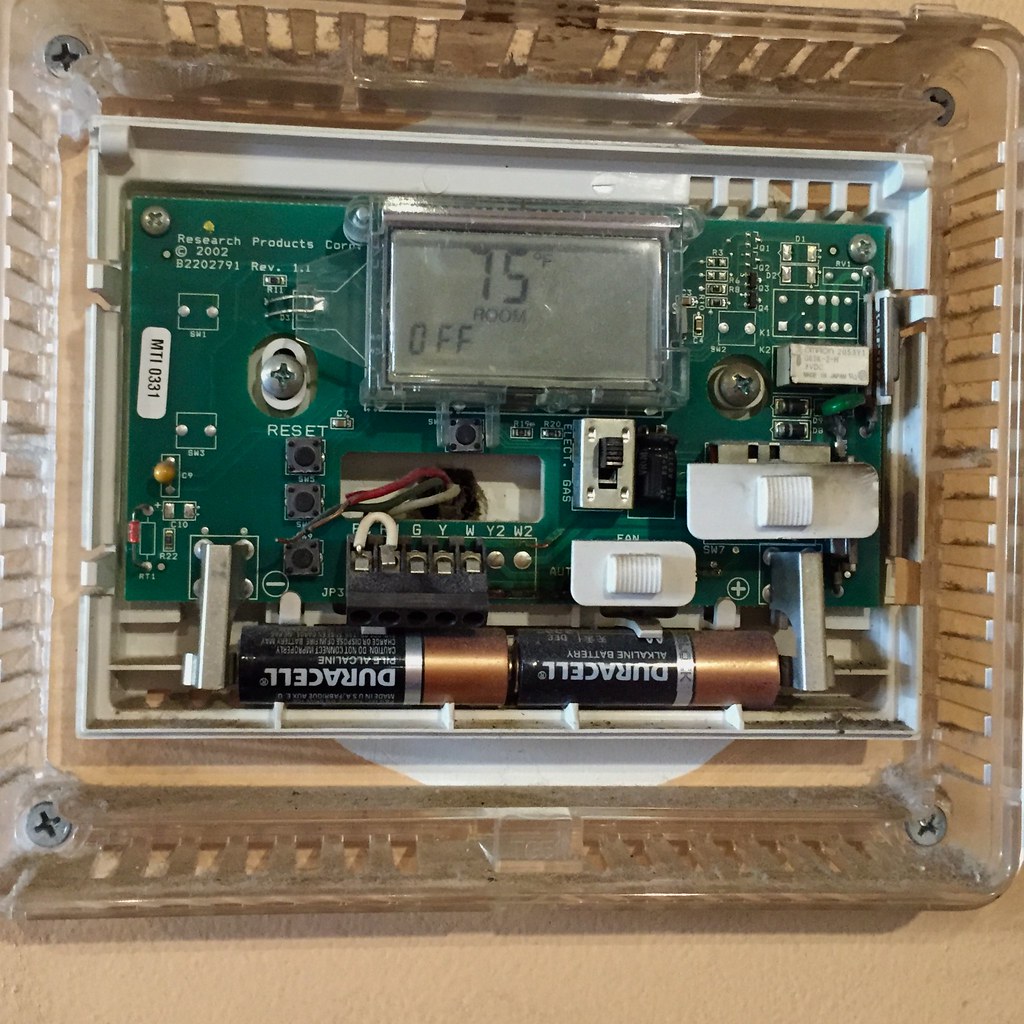This aerial photograph captures the intricate interior mechanism of a thermostat, enclosed within a dirty, clear plastic square casing secured by screws at each corner for wall attachment. Central to the composition is a green circuit board housing various small electronic components. Two cylindrical batteries are prominently nestled within the unit. The board also features a distinctive black switch set against a chrome background, alongside two white texturized switches. Three wires—colored red, blue, and white—are visibly connected, suggesting their role in the device's functionality. A transparent section of the plastic casing clearly displays the temperature reading of 75 degrees Fahrenheit, as well as labels for room and off settings. This image provides a detailed glimpse into the essential workings of a home thermostat.